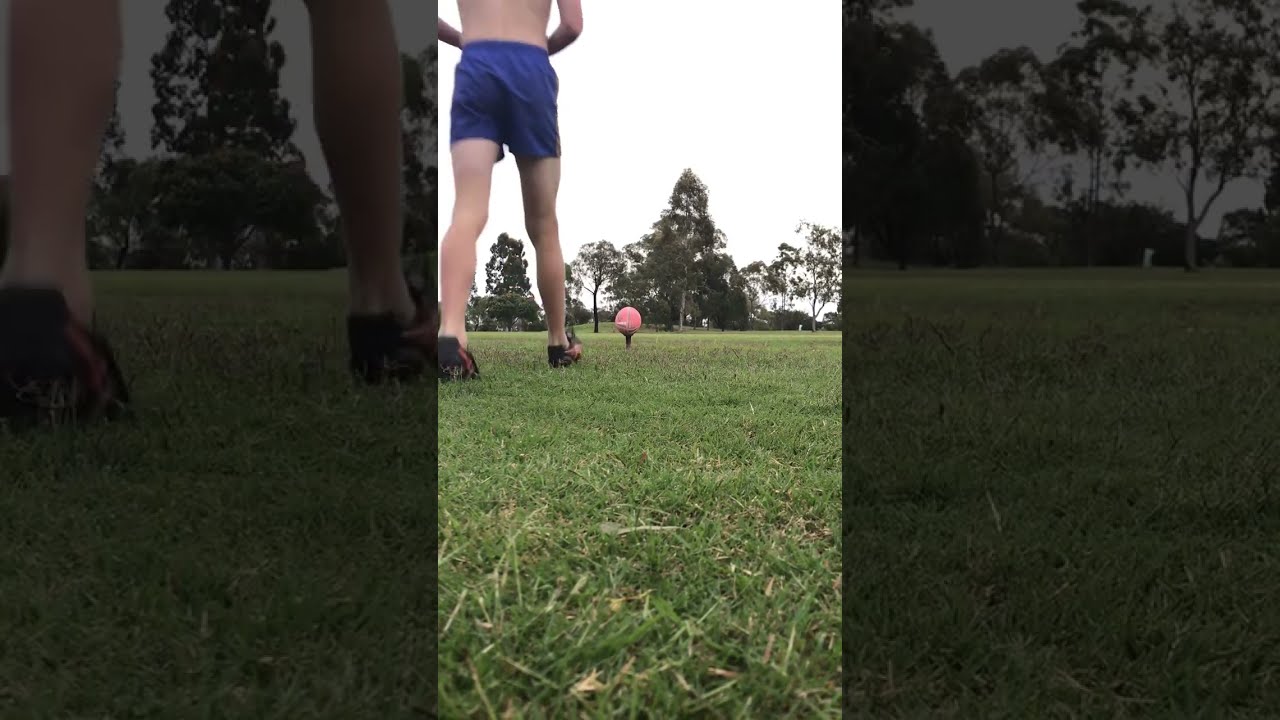In the foreground of this vertically oriented cell phone image, a shirtless man is captured from behind, standing on a neatly trimmed grass field with a bright gray sky overhead. Dressed only in blue athletic shorts and reddish-orange shoes, he appears to be lining up for a kick. A red ball, possibly a rugby ball, rests flat on a non-typical tee just a few feet in front of him. The camera is positioned low, just inches from the ground, offering a direct view along the field's surface with trees forming a distant border approximately 400 meters away. The image is taken in broad daylight with the man positioned slightly to the upper left, walking towards the ball, emphasizing his athletic build. The background complements the main image with zoomed-in, faded duplicates of the scene on either side.